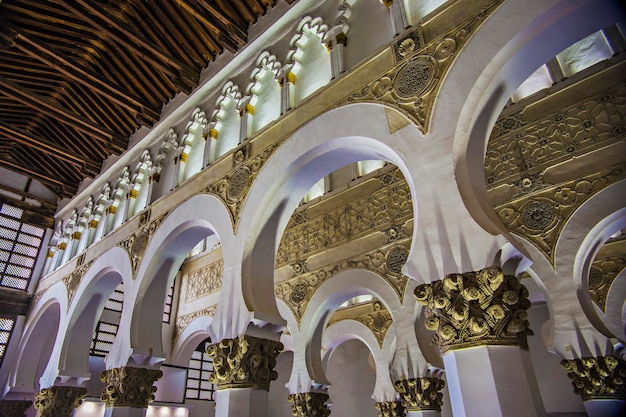The image captures the interior of a grand and ornate public building, likely a historic church or cathedral. The photograph is tipped upwards, showcasing the ceiling and a portion of the upper walls. The ceiling features dark wooden beams that intersect horizontally and vertically, creating a distinctive triangular point running from the back left to the front right. The arches, which repeat identically from left to right, are crafted from white marble stone with elaborate gold detailing. The vertical parts of these arches are intricately adorned, with gold filigree and relief artwork adding to the magnificence. 

Between the arches, the back wall is richly covered in gold leaf, featuring detailed carvings etched into the surface. The decorative columns supporting these arches have highly ornate gold upper portions, and a series of round, wave-like designs extend towards the ceiling, creating a layered visual impression. The warm lighting enhances the gold detailing, suggesting either natural light filtering through tinted windows or artificial uplighting from below. 

Additionally, the far left side of the image hints at a series of horizontal, rectangular window panes, adding to the overall grandeur. The combination of white, gold, and dark brown hues, along with the detailed ornamentation, emphasizes the building's historic and majestic ambiance.